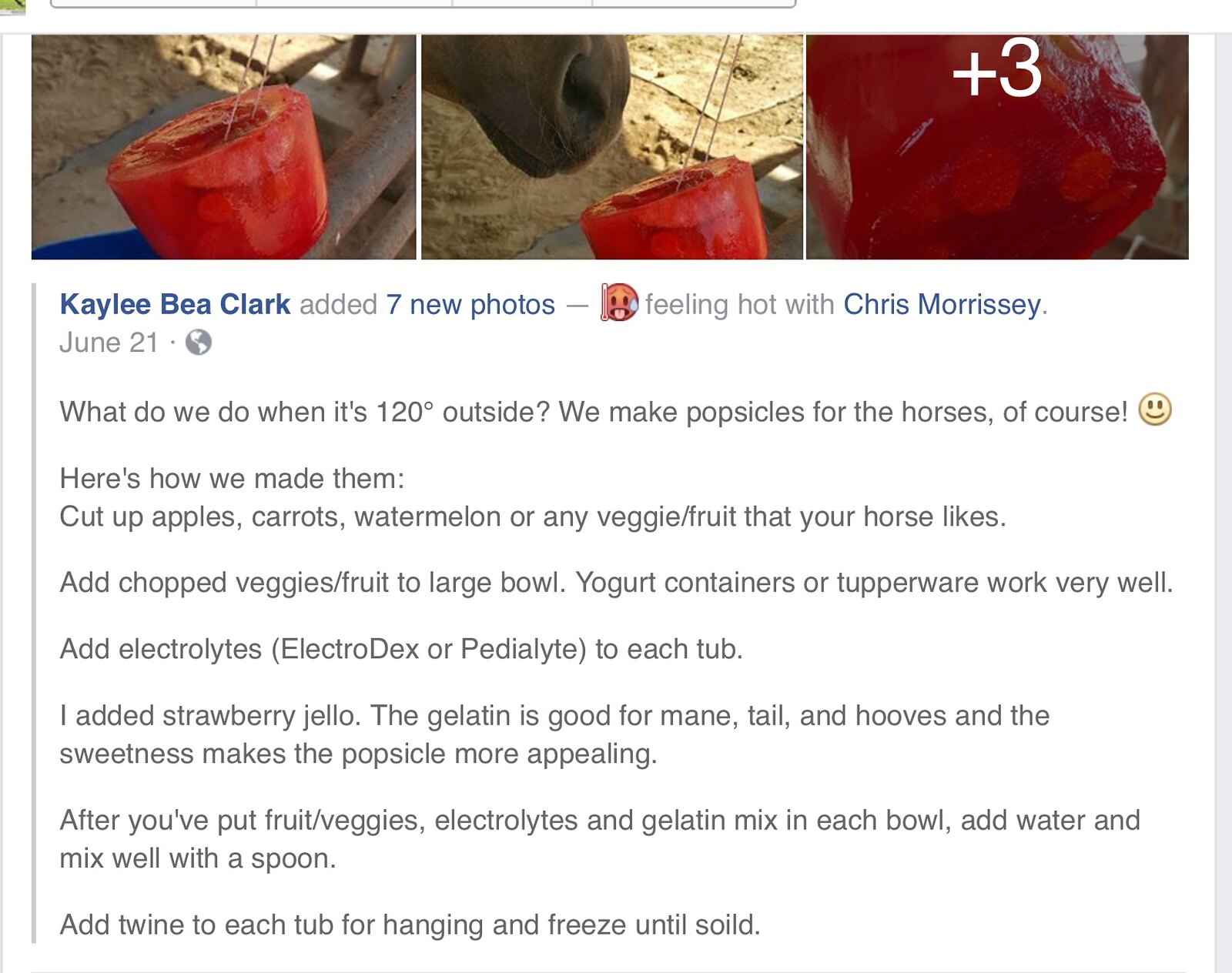The image appears to be a screenshot of a Facebook post made by Kaylee B. Clark on June 21st, documenting the process of making popsicles for horses to keep them cool during extreme heat. The post is set to public and mentions feeling hot with Chris Morrissey. At the top of the image, there are three pictures, with the third stating "plus three," indicating additional images can be viewed. The pictures show close-ups of the homemade horse popsicles, composed of chopped apples, carrots, watermelon, and other fruits and veggies mixed with electrolytes or strawberry Jello and frozen with twine attached for hanging. The middle image partially displays the muzzle of a horse approaching the treat. The detailed recipe included in the post explains the preparation steps for these refreshing popsicles against a background of blue, dark blue, black, and white, with accents of brown and red.